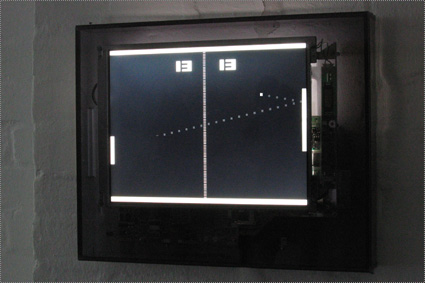The image depicts a flat-screen monitor mounted on a gray stone or white brick wall. On the screen, there's a classic video game, Pong, in progress. The display features a predominantly black background with a vertical white line in the center, representing the middle of the playing field. On either side of this vertical line are two rectangular white paddles, one on the left and one on the right, positioned to return a bouncing ball—a small white dot seen near the middle of the screen. The paddles and the ball are situated among dotted lines forming a boundary. At the top of the screen, the score is visible, with both players tied at 13 points each. The monitor is enclosed in a black plastic border, providing a clear and classic view of this vintage game.